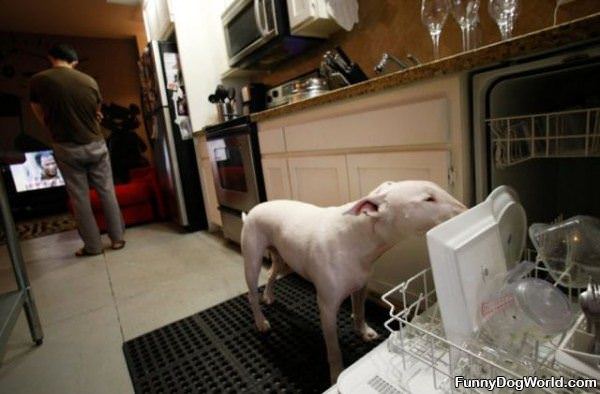In a cozy kitchen scene, a pinkish-white dog, with short ears and short hair, stands on a brown mat in front of the sink, diligently licking a large white plate inside an open dishwasher. The dog’s eye and the side of its face are visible, though its mouth and nose are hidden behind the plate. Dirty dishes fill the bottom rack of the dishwasher, while empty wine glasses rest on the counter above. The kitchen features large white square tiles on the floor and white cupboards with matching drawers. In the background to the left, a dark-haired man in jeans and a green or brown t-shirt is standing barefoot, looking towards a TV in the living room, his posture suggesting he might be holding something or simply watching the screen.